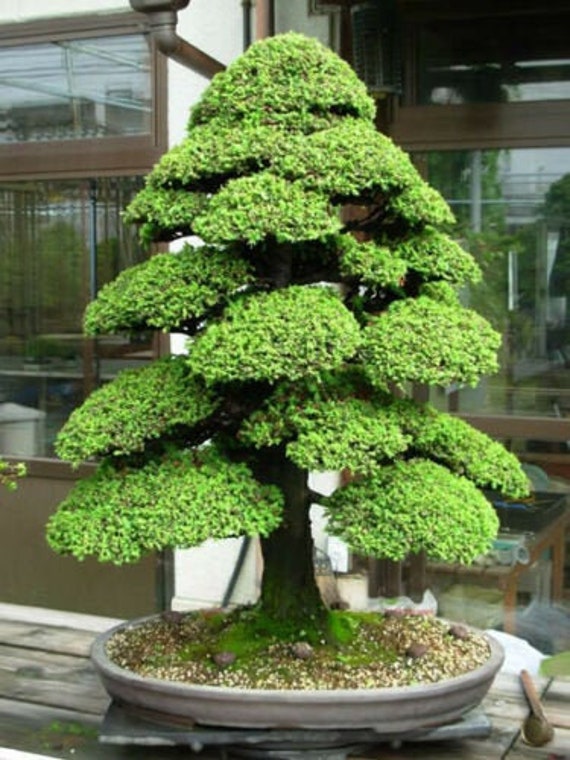This image showcases a captivating bonsai tree, somewhat larger than a typical bonsai, with a distinct Christmas tree shape. The tree resides in a shallow, oval bonsai pot, characteristic of bonsai culture, adorned with moss and rocks at its base. Its branches, clothed in luxuriant, algae-textured leaves, form lush, triangular pads that taper towards the top, culminating in a verdant dome. The trunk is a natural brown, contrasting with the vibrant green of the foliage. The scene is set outdoors in a courtyard, positioned on a wooden table with vertically aligned slats. The background reveals a building featuring white and brown sections, multiple windows, a foosball table visible inside, and a brown irrigation pipe leading to a concrete circle below. The lack of people suggests a serene, unoccupied space, possibly outside a restaurant.